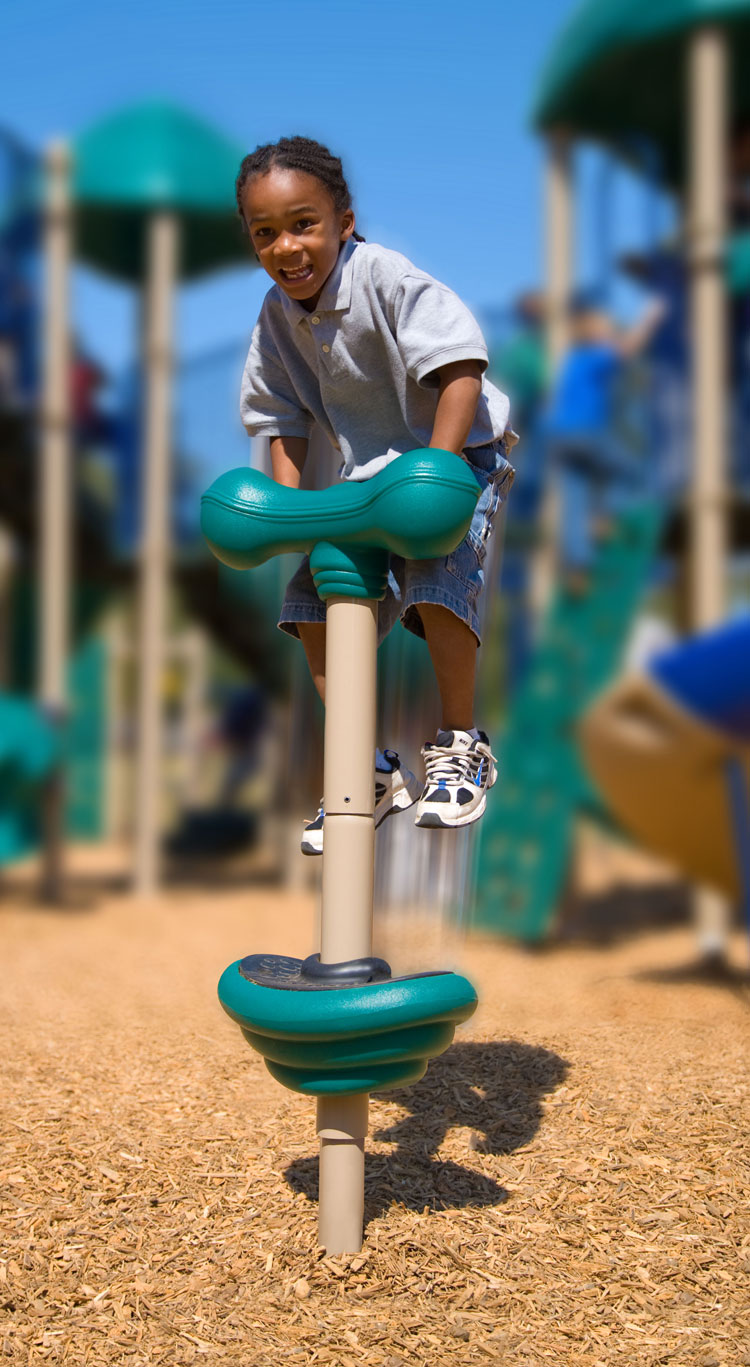This outdoor color photograph captures a joyful African American child, approximately four years old, playing on a playground. The child, sporting dreadlocks and a radiant smile, is dressed in a gray polo shirt, blue jean shorts, and white tennis shoes. He is energetically climbing onto a green playground structure, equipped with a wider top seat and a broad bottom, supported by a brown pole. The ground beneath is covered in brown wood shavings, providing a soft landing surface. In the blurred background, additional playground equipment, including slides and a jungle gym, can be seen, predominantly in shades of green and brown. The lighting suggests a sunny day, casting a short shadow of the child on the ground. The scene exudes happiness and the carefree spirit of childhood.